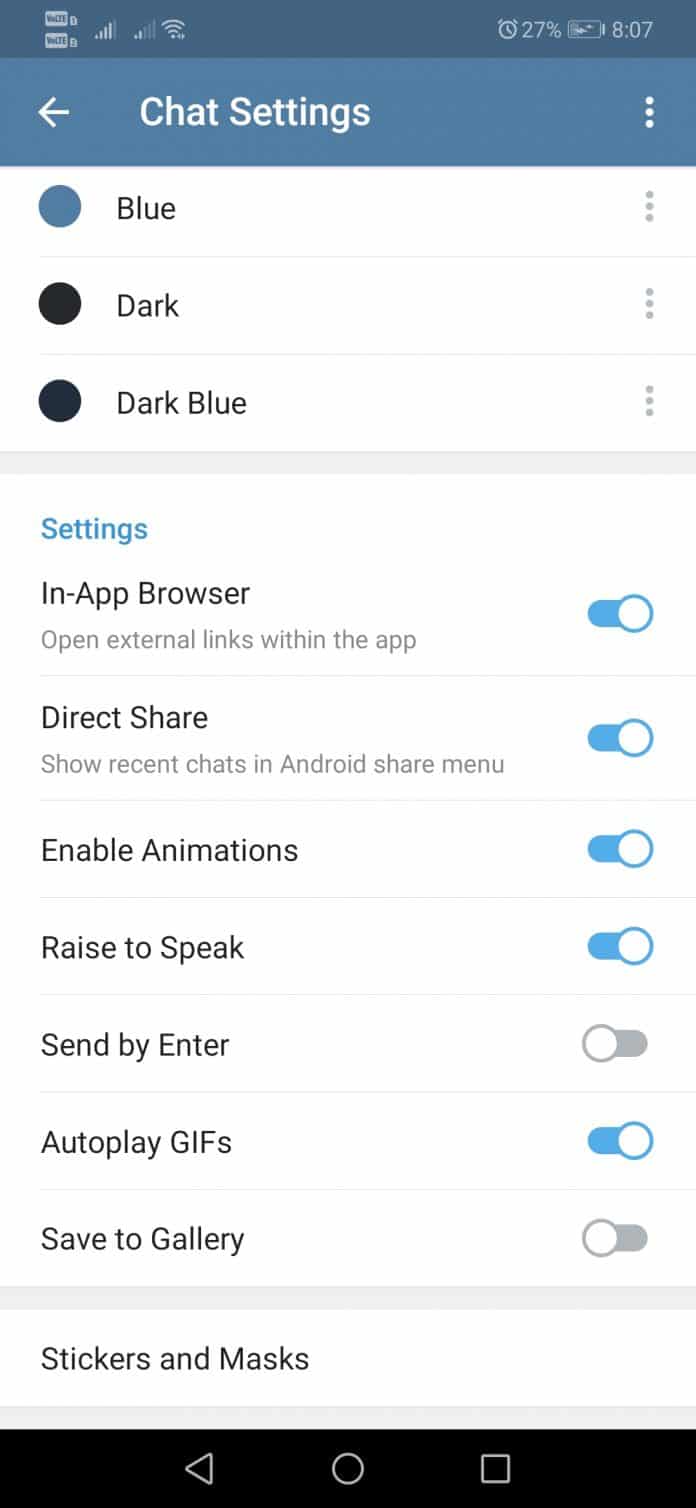The image is a screenshot of a cell phone, showcasing various interface details and settings. 

In the upper left-hand corner, there are two cell phone reception icons, one indicating four bars of signal strength while the other shows two bars. Adjacent to these is a Wi-Fi icon, which displays full strength. 

The upper right-hand corner reveals the time, marked at 8:07, alongside a battery icon showing a 27% charge. An alert icon, signaling a reminder or alarm, is also visible.

Centered below these indicators is the header titled "Chat Settings." Under this heading, there is a section displaying three color options: "Blue," "Dark," and "Dark Blue." Each option is accompanied by a corresponding circular icon on the left—blue has a blue circle, dark has a black circle, and dark blue has a dark blue circle.

Further down, there is an array of toggle settings:
- "In-app browser" is toggled on.
- "Direct Share" is toggled on.
- "Enable animations" is toggled on.
- "Raise to speak" is toggled on.
- "Send by Enter" is toggled off.
- "Autoplay GIFs" is toggled on.
- "Save to gallery" is toggled off.

The screenshot captures a detailed view of various connectivity statuses, battery life, time, and specific user settings within a chat application.